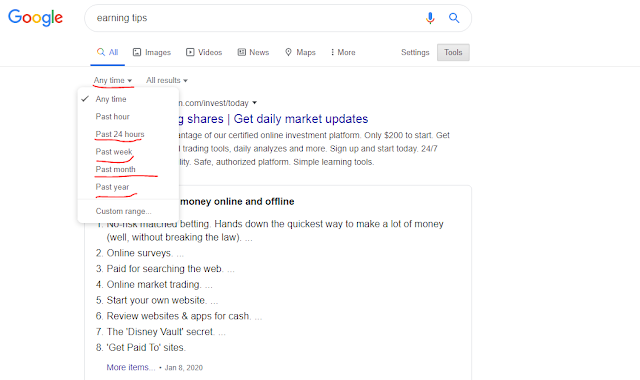This image, dated January 8, 2020, appears to be sourced from a website, possibly Google, that discusses various ways to earn money. The text on the image lists several methods in a detailed format, highlighting:

1. No Risk Matched Betting: Described as a highly lucrative method to earn substantial money without any legal risks.
2. Online Surveys: Participating in surveys for financial compensation.
3. Paid for Searching the Web: Earning money by simply searching online.
4. Online Market Trading: Investing and trading in online markets to generate income.
5. Start Your Own Website: Launching a personal website as a potential revenue stream.
6. Review Websites and Apps for Cash: Getting compensated for critiquing websites and applications.
7. The Disney Vault Secret: Likely hinting at a strategy involving buying and selling Disney merchandise or media.
8. Get Paid to Sites: Engaging with websites that pay users for various activities.

There's also a link provided for accessing more ways to earn money, indicating that the content continues beyond what is listed.